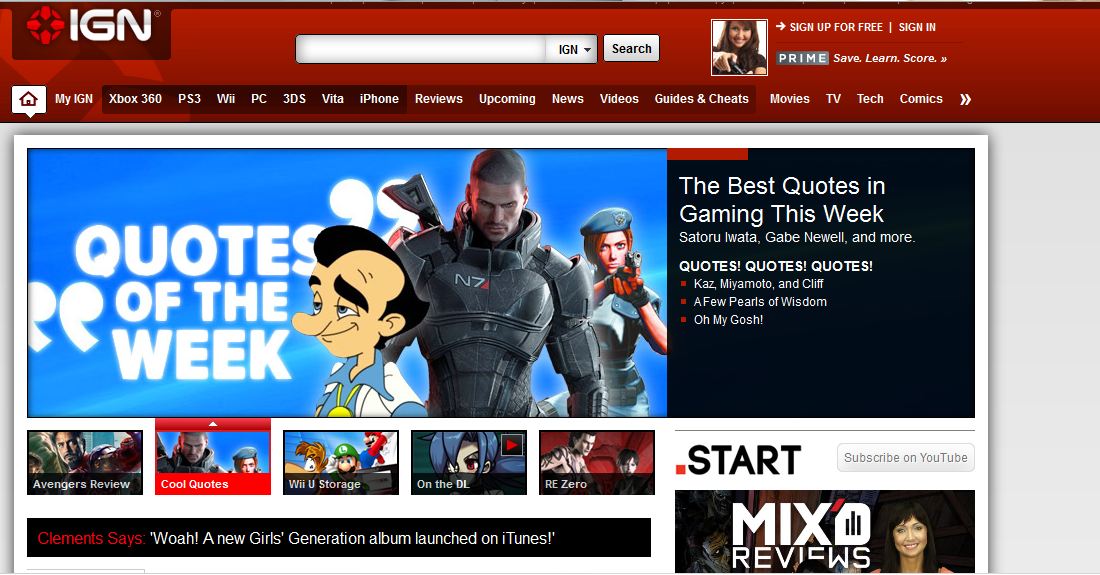This image is a detailed snapshot taken from the popular gaming website IGN. The website's title and iconic red logo are prominently displayed in the top left-hand corner on a bright red banner. This banner also features various navigational categories and buttons that provide access to different sections of the website. These categories include Xbox 360, PS3, Wii, PC, Nintendo 3DS, PS Vita, iPhone, reviews, upcoming products, news, videos, and guides and cheats.

Centrally positioned on the webpage are three distinct video game characters. The first character appears to be a cartoon figure of a man looking towards the left. The second character is depicted as a heavily armored soldier or warrior. The third character is a woman who seems to be a police officer; she is holding a gun and pointing it forward, as if shooting at something.

Below this central image, there are additional clickable sections with intriguing titles such as "Avengers Review," "Cool Quotes," and "Wii U Storage." These sections likely lead to specific articles or content related to the respective topics. The entire layout is designed to engage users and provide easy access to a wide range of gaming-related information and content.